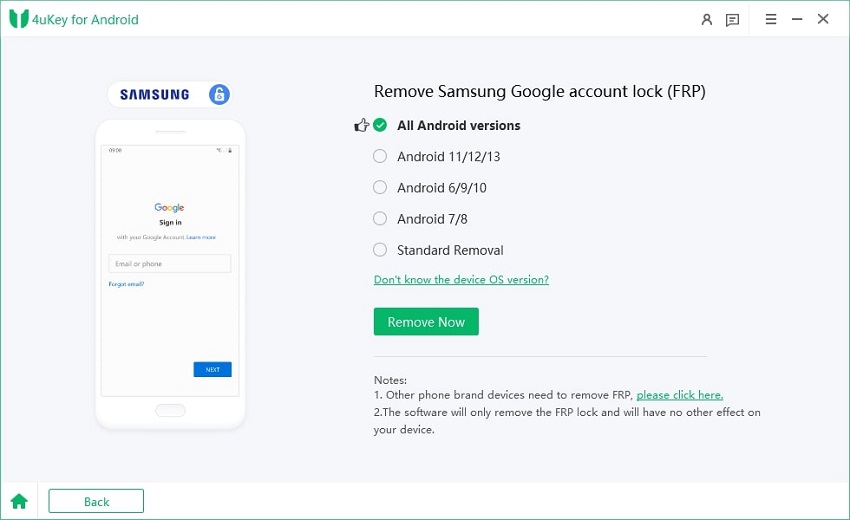An image showcasing the 4uKey for Android interface. At the top, a white bar displays the green 4uKey for Android logo. The top-right corner features user, chat, and several other icons. Below, a gray block spans the bottom section of the image. On the left side of this block, there is a Samsung icon with a lock symbol beside it. Adjacent to it, a white mobile device screen showing the Google sign-in page with an address bar for email or phone number and a blue "Next" button is displayed. To the right of the mobile device, text reads: "Remove Samsung Google account lock (FRP) - All Android versions." Below this, a button labeled "Remove Now" is present. The bottom section includes two notes with hyperlinks for other phone brands. The bottom left corner contains a home button and a back button.